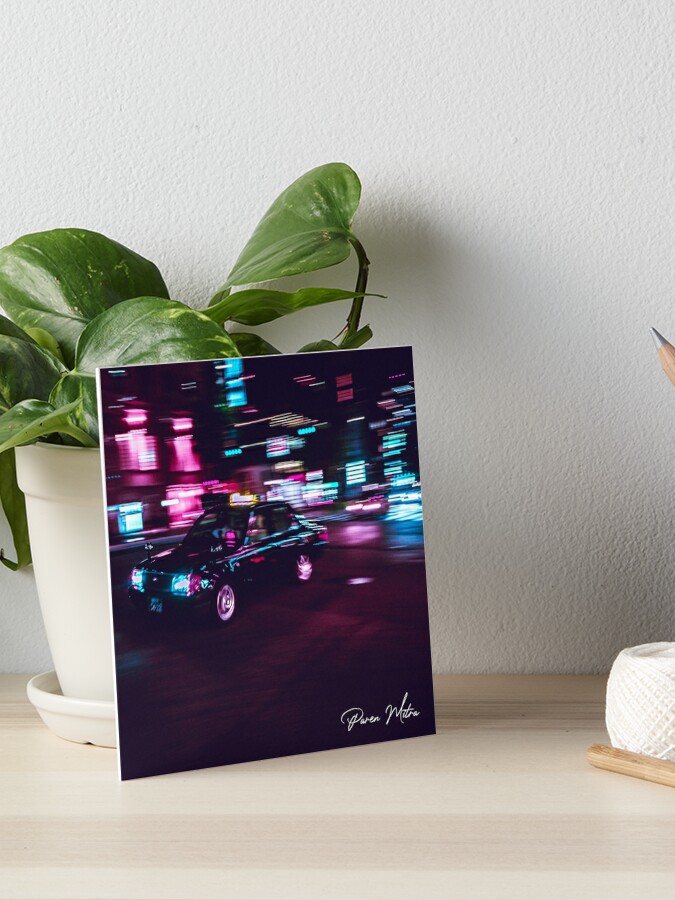The image depicts a framed print leaned up against a white flower pot containing a lush green plant with large leaves. The artwork, signed in the bottom right corner, features a black European taxi car speeding through a bustling city street at night. The cityscape around the car is filled with vibrant neon colors, predominantly blue and purple lights, adding a sense of motion and energy to the scene. The image is slightly blurred, emphasizing the car’s speed as it reflects the city lights. Resting on a wooden table, the print shares space with a small package of string and the tip of a pencil, adding to the still-life composition. The background showcases a white textured wall, providing contrast to the vivid artwork and enhancing the overall aesthetic.